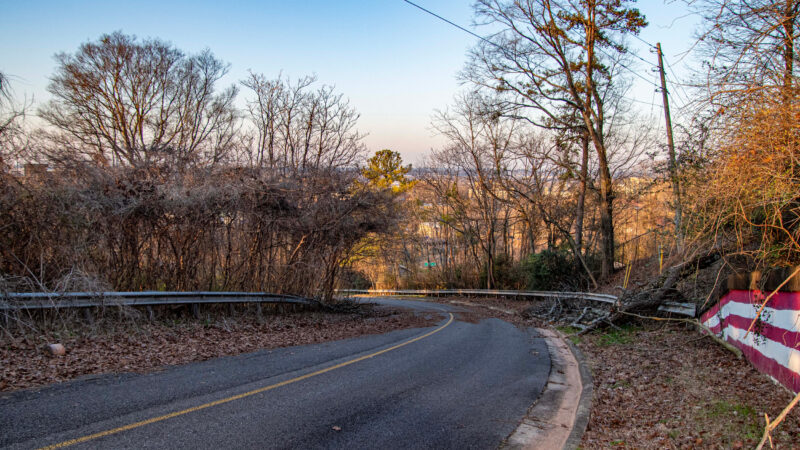The image depicts a winding road situated in a hilly or mountainous forest area during the late fall or early winter season. The road, which curves sharply to the left with a blind turn, is bordered by metal guardrails on both sides and marked with a single yellow line in the middle. The surrounding trees are mostly leafless, indicative of the winter season, with fallen leaves and brush accumulating along the edges of the road. A large branch has fallen over the guardrail on the right side. A concrete wall with red and white stripes is also visible on the right, possibly serving as a retainer or barrier. There is a telephone wire stretching across the road from a pole positioned on the right side. In the distance, hints of a town or city can be glimpsed through the trees, and a delicate turquoise hue is also noticeable among the foliage. The overall atmosphere suggests a quiet, somewhat desolate natural setting with nature beginning to reclaim the area.